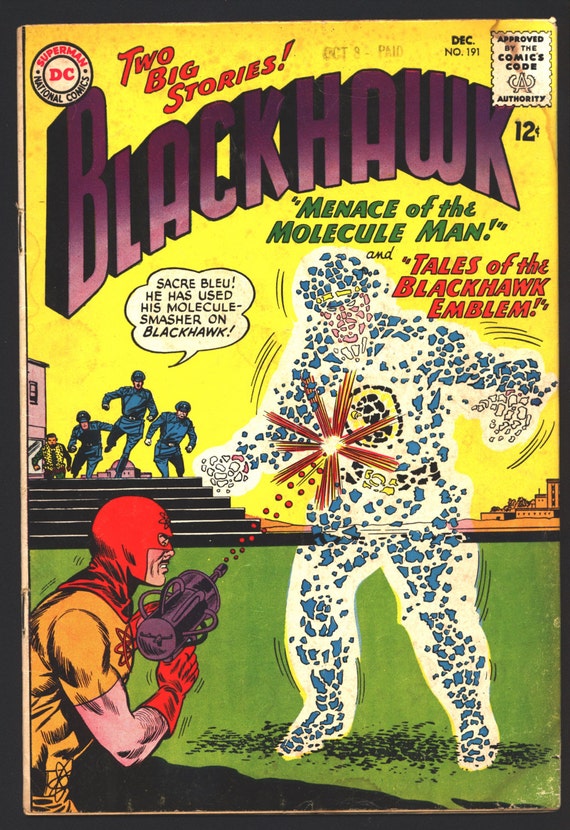This image is a scan of a brilliantly illustrated comic book cover, presented in a portrait style. The cover is predominantly yellow, featuring a yellow sky that melds into an orange city skyline, casting a striking light across the horizon. Below this dynamic skyline is a patch of green grass, adding a touch of nature to the urban backdrop.

The main title of the comic book, "Black Hawk," is rendered in a curved, violet text with a dramatic black shadow that makes it stand out against the colorful background. The cover also boasts the iconic DC logo, a round emblem inscribed with "DC" at the center and encircled by the words "Superman" and "National Comics."

Above the title "Black Hawk," a bold headline in red text announces, "Two Big Stories," creating an immediate sense of excitement. Below the title, the issue's main feature is highlighted in quotes: "The Menace of the Molecule Man."

The illustration is action-packed, depicting a man with a red mask firing a weapon at another man, who appears to be disintegrating into fragments. As this intense scene unfolds, four people are seen running towards the action, one of them exclaiming in a word balloon, "Sacre Bleu! He used his Molecule Smasher on Black Hawk."

Beneath the main feature title, smaller text introduces "Tales of the Black Hawk" in bold red letters, adding further intrigue to the compelling cover. The overall composition of the cover skillfully blends vivid colors, dynamic text, and dramatic action, capturing the essence of a classic comic book adventure.